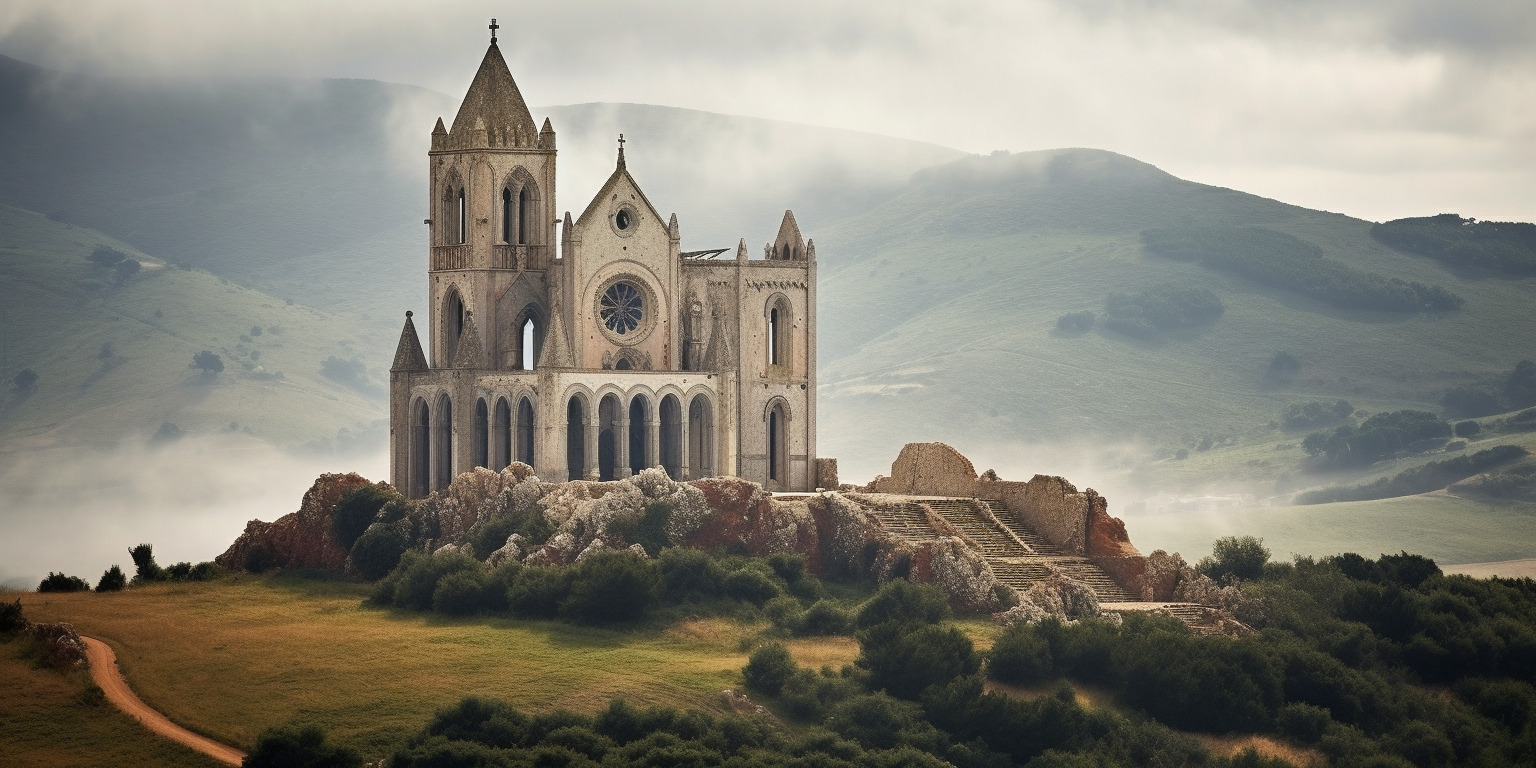The image depicts a detailed and captivating illustration, possibly animated, of an ancient and majestic castle or cathedral nestled in a lush valley. The foreground is replete with a variety of colorful shrubbery, including greens, whites, and reds, which lend a dynamic and vibrant feel to the scene. The castle, constructed from white stone, boasts several spires and peaked areas, and its architecture features arched windows and columned, arching entrances, reflecting an old-world charm. The edifice is set atop a series of worn, concrete steps that indicate its age, hinting at a history of grandeur now faded. Behind the castle, rolling green foothills, almost mountainous but smooth, rise up amidst a thick blanket of fog that descends to the ground, creating a mystical atmosphere. A small dirt path or walkway snakes along the left side of the image, emphasizing the enormous scale of the castle and suggesting that it might serve as a sightseeing or tourist spot today. Despite the ruinous aspects, such as crumbling walls and deteriorating stairs, the picture conveys a sense of timeless beauty and historical intrigue.